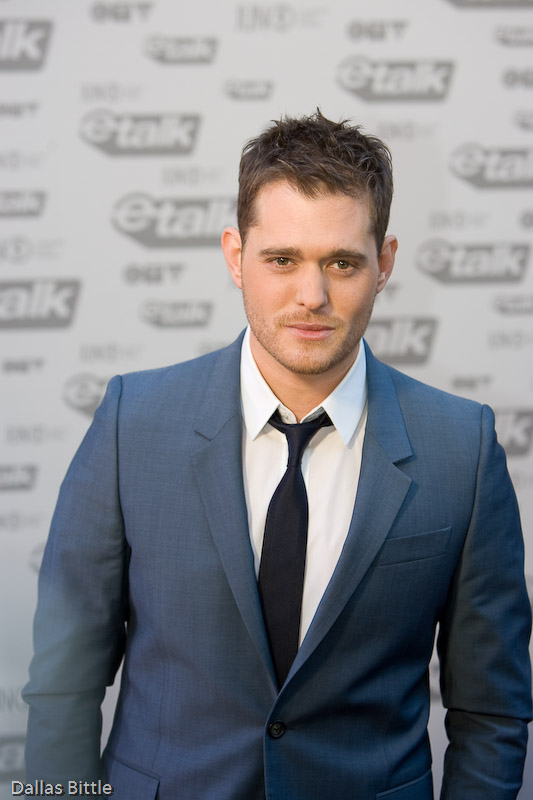The image is a color photograph of singer Michael Bublé, who appears to be the main subject. He is dressed in a medium-toned grayish-blue suit paired with a dark blue or light black tie and a white button-down shirt. His hair is dark brown, spiky, and slightly messy, and he sports a five o'clock shadow, with brown eyebrows and brown eyes. Bublé is smiling subtly, standing with his arms at his sides, and looks slightly off-guard, suggesting this may be a professional paparazzi shot taken at an event.

In the background, there is a prominent white sign with the name "e-talk" repeated in gray logos. The only other visible text in the bottom left corner reads "Dallas Biddle." The colors in the image include tones of black, white, brown, dark bluish-gray, peach, and pink, contributing to the overall professional ambiance of the event.